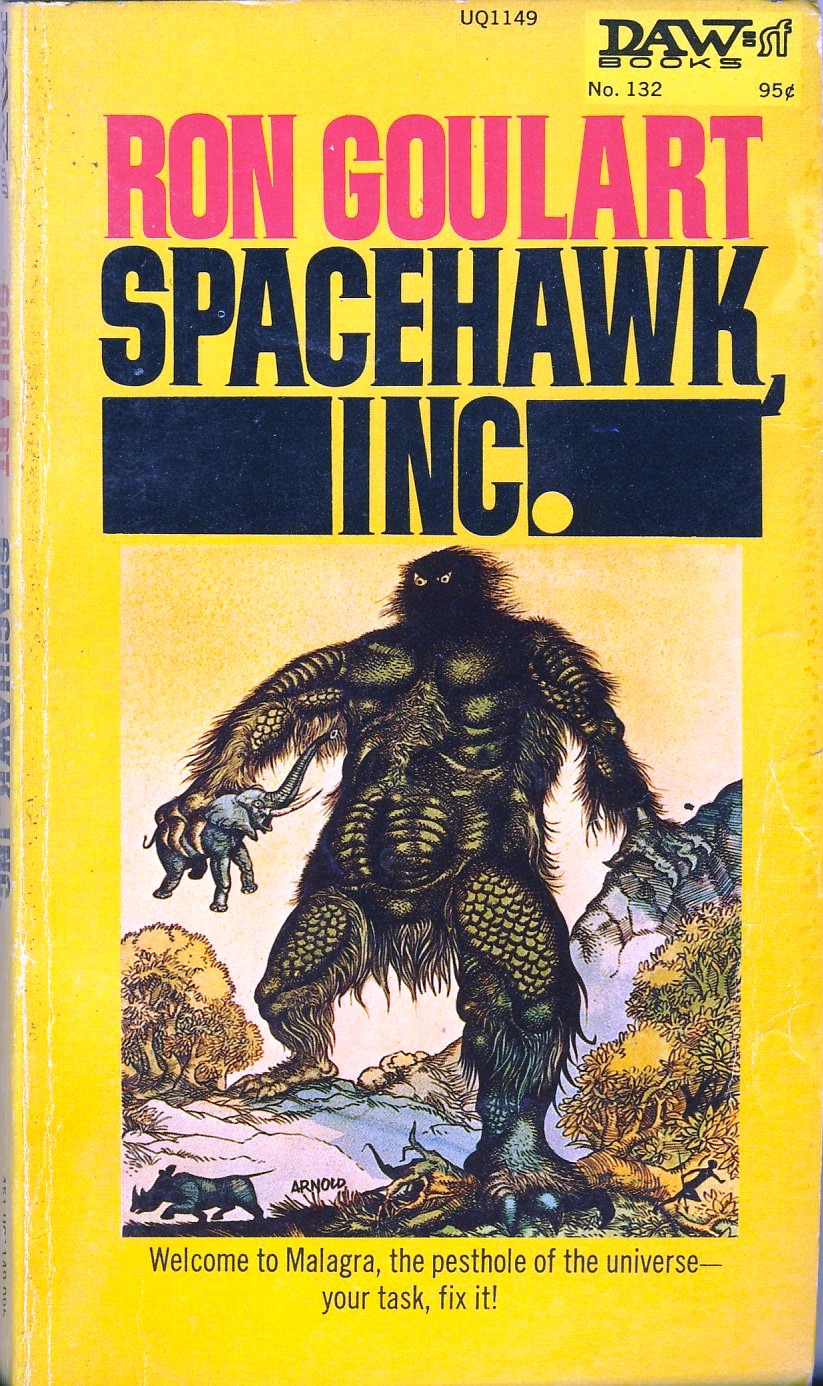This image depicts the cover of a science fiction paperback book titled "Space Hawk, Inc." by Ron Goulart, published by Doa Books as number 132 and priced at 95 cents. The background is a vivid yellow, with the author’s name, Ron Goulart, in bold pink text at the top. Below the author’s name, the book title, "Space Hawk, Inc.," is displayed in black letters. The upper right corner features the letters "SF," indicating the book's science fiction genre.

Dominating the cover is a detailed color illustration of a towering, fearsome monster with both furry and scaly features, white eyes, and looking to the left. The creature, with light green scales on its arms and legs, holds an elephant in its right hand, emphasizing its immense size. At the bottom left of the illustration, a rhinoceros is seen running, and another rhinoceros seems to be crushed under the monster's feet. The background features trees and rocky, hilly terrain, with the monster overshadowing the landscape.

The bottom of the cover includes the ominous tagline in black text: "Welcome to Malagra, the pest hole of the universe. Your task, fix it." The illustration is attributed to an artist with the last name Arnold.